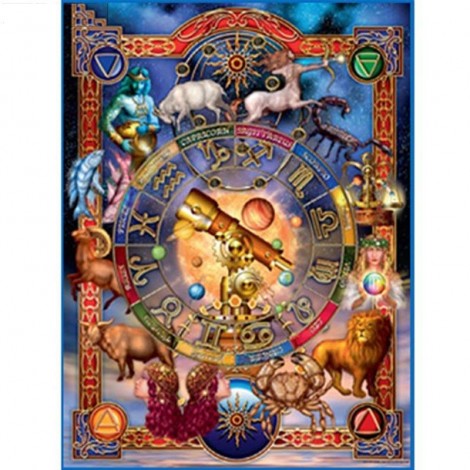The image depicts the back of a tarot card designed with a richly detailed and colorful celestial theme. The background features a deep blue sky adorned with clouds and stars, creating a dreamlike, cosmic atmosphere. Central to the design is a circular motif encompassing the 12 zodiac signs, each labeled with their respective symbols. Surrounding the circle are vivid illustrations of various celestial and mythological figures, including a lion for Leo, a crab for Cancer, a bull for Taurus, a ram for Aries, a pair of fish for Pisces, and a scorpion for Scorpio. There are also representations of other signs, such as a centaur for Sagittarius and a minotaur-like figure. The circle itself is segmented into arcs of red, blue, yellow, and green, giving it a vibrant, rainbow-like appearance. Additionally, the center of the circle features a telescope pointed towards the top left, with intricate golden gears and planets in the background, reinforcing the celestial theme. The entire scene is framed by a striking red border, with corners adorned with multicolored triangles, adding to the complexity and vividness of the illustration. The design culminates in a visually stunning and intricate portrayal of the zodiac within a fantastical, starry universe.